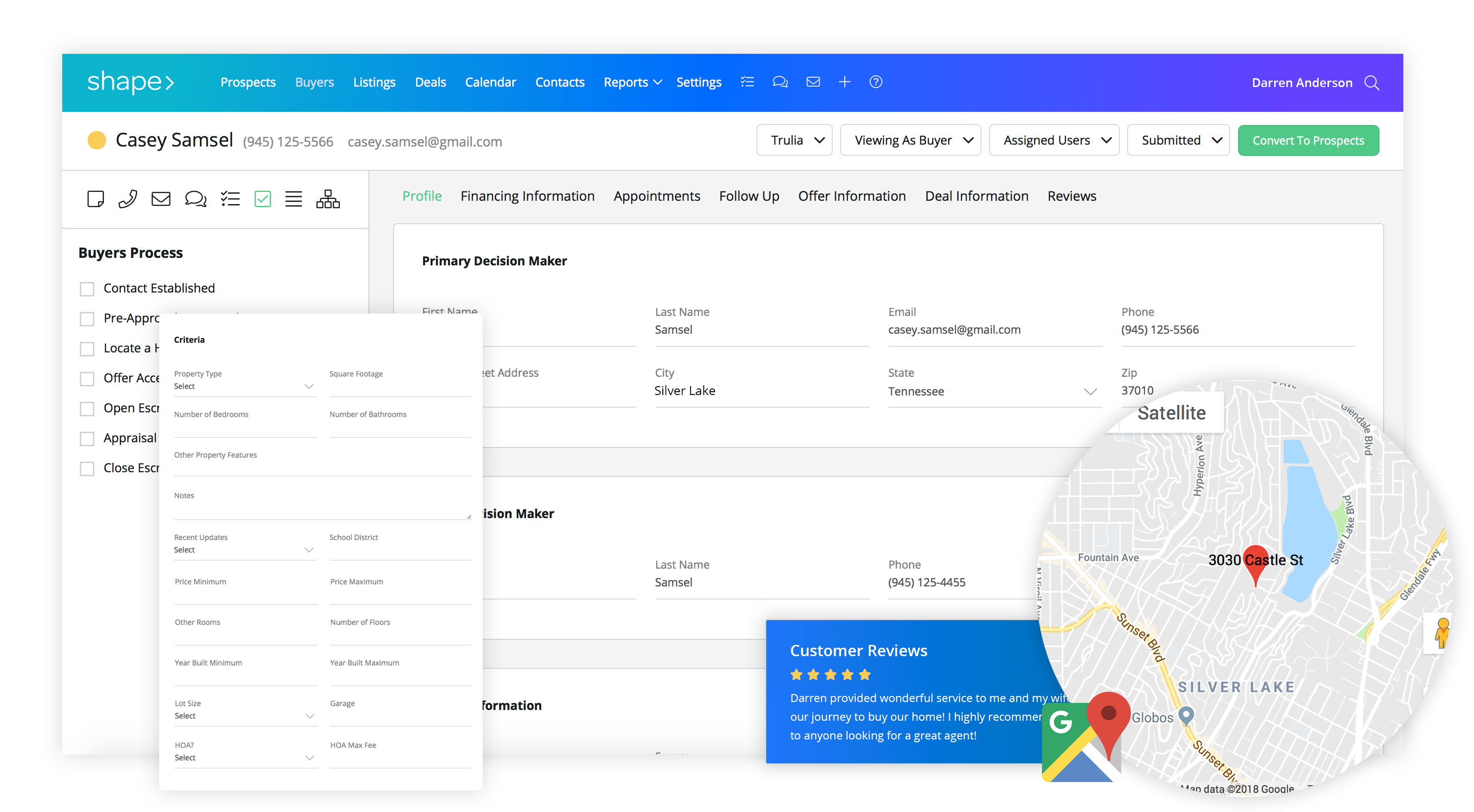This image is a screenshot of a program interface displayed on a computer. The layout is a rectangular shape, wider than it is tall. The interface features a prominent top banner, transitioning from turquoise to a dark bluish-purple gradient. In the upper left-hand corner, a logo shaped like an icon is visible, followed by several drop-down menu tabs labeled: Projects, Buyers, Listings, Deals, Calendar, Contacts, Reports, and Settings.

In the upper right-hand corner, the logged-in user is identified as Darren Anderson. The primary section below the gradient banner showcases a white rectangular area where a yellow circle icon precedes the name "Casey Samuel," alongside a telephone number and an email address, suggesting a customer database interface.

The principal window offers various selectable categories such as Profile, Financing Information, Appointments, Follow-up, Offer Information, Deal Information, and Reviews. At present, the 'Profile' section is selected, displaying detailed information like contact data, mailing address, decision-maker details, among other specifics.

On the left side of the interface, a toolbar lists different buyer process checklists available for selection. Additionally, in the bottom right corner, there's a circular map pinpointing Casey Samuel's location in Silver Lake, Tennessee.